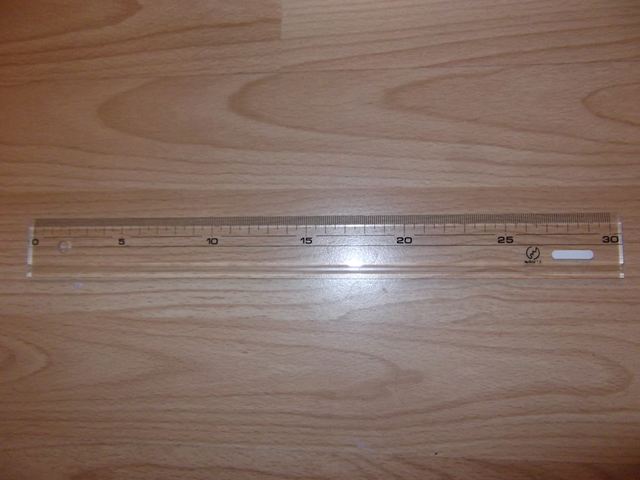The image showcases a transparent plastic ruler placed on a light, possibly artificial wood surface with a wide, unstained grain pattern. The ruler, which has a hole near the center of the left end, starts its measurements at zero and is marked in increments of five, from 0 to 30. Each major interval is subdivided into ten smaller divisions. A small, round logo featuring a diagonal zigzag design is present on the ruler, although the text is too small to discern even on zoom. A bright glare is visible on the ruler between the 15 and 20 marks, caused by a light source reflecting off its surface.